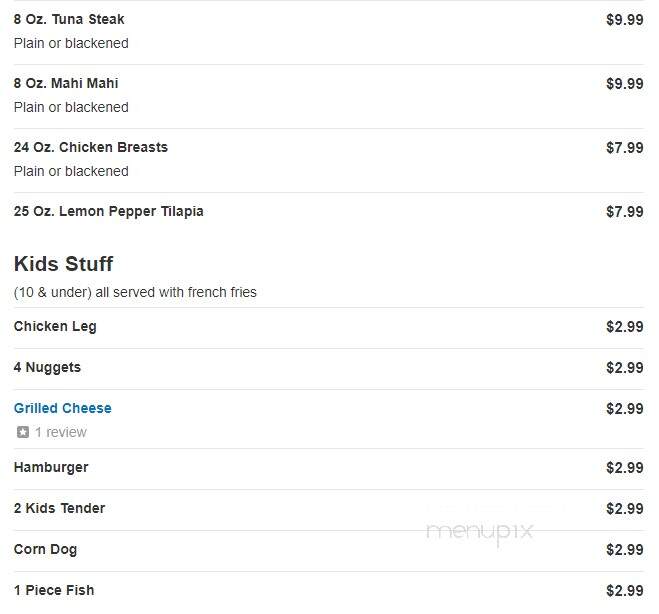**Detailed Caption:**

This image is a screenshot of a menu, likely sourced from a platform named "MenuPix," as indicated by the watermark at the bottom of the image. The menu is organized into a vertical column with the food item names on the left and their corresponding prices on the right, creating a clear and legible layout. 

At the top section of the menu, it features various seafood and poultry options: an 8-ounce Tuna Steak, available plain or blackened, priced at $9.99; an 8-ounce Mahi-Mahi, also available plain or blackened, for $9.99; a 24-ounce Chicken Breast, which can be ordered plain or blackened, costing $7.99; and a 25-ounce Lemon Pepper Tilapia, priced at $7.99.

The lower section of the menu is dedicated to "Kid's Stuff," indicated in bold letters with a note specifying that these items are for children 10 years and under, all served with French fries. The kids' options include a Chicken Leg for $2.99, Four Nuggets for $2.99, and Grilled Cheese, listed in a blue font and noted to have one review, also at $2.99. Additionally, other kids' items available for $2.99 each are: Hamburger, Two Kids' Tenders, Corn Dog, and One Piece Fish.

The appearance of the menu suggests it is electronic, as there is no logo of the restaurant visible in the screenshot.